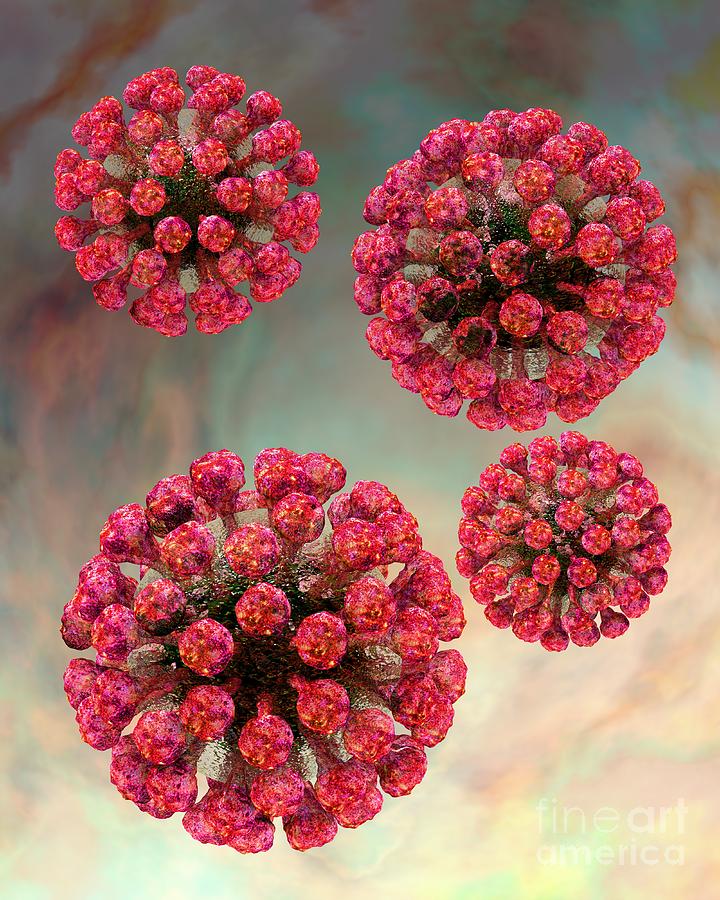The image is a detailed, computer-generated illustration of four identical, spherical structures resembling a virus or chemical molecule. Each structure features a dark core - black or dark brown - with numerous red appendages radiating outwards, reminiscent of lollipops or mushrooms with yellow dots. These formations are situated against a dynamic background that transitions from a dark black at the top to a bright, oil-slick of shimmering white, green, and pink towards the bottom right-hand corner. Positioned differently in size, the largest sphere is at the bottom left, followed by a slightly smaller one at the top right, another smaller yet at the top left, and the smallest at the bottom right. The background's interplay of colors, including blue, gray, tan, pink, and green, enhances the contrast against the uniformity and vibrant detail of the spherical structures.